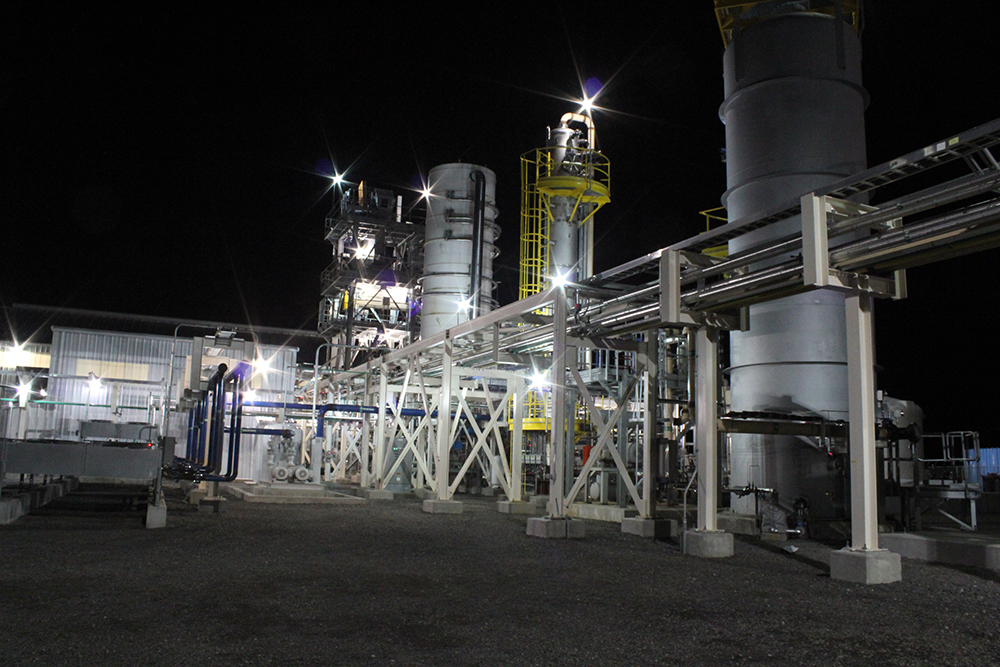This nighttime photograph captures an expansive industrial yard bustling with colossal machinery and structures, possibly involved in power generation or heavy industrial processes. The scene is vividly illuminated with bright, scattered lights that create a stark contrast against the dark night sky. Yellow staircases and ladders stand out prominently among the gray and white steel beams and piping that cover the area. Central to the image is a brightly lit, yellow catwalk that crosses over a section of the complex, resembling a bridge.

The ground appears to be covered in gravel, adding texture to the scene. On the left side, there's a rectangular silver building with additional smaller metallic structures and windows nearby. Blue shipping containers add a touch of color to the background. Moving towards the center-right, the yard features several circular steel towers and tubes, along with white and gray cylindrical buildings equipped with various pipes. These structures seem to be interconnected by the pervasive network of industrial piping and steel supports.

Overall, the image evokes a sense of organized complexity, where each element — from the towering steel frameworks to the small, scattered lights — contributes to the dynamic and industrious atmosphere of the yard.